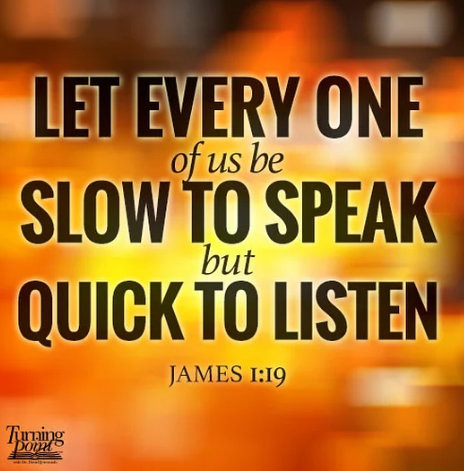The image is a small square with a vibrant, abstract background that resembles blurred flames, blending oranges, yellows, and whites with a touch of blacks and grays at the top. The central text, derived from the Bible, prominently features the quote "LET EVERYONE OF US BE SLOW TO SPEAK BUT QUICK TO LISTEN," with certain words ("LET EVERYONE," "SLOW TO SPEAK," and "QUICK TO LISTEN") in large, bold, black capital letters, while "of us be" and "but" are in a smaller, thinner font. At the bottom left corner, there is a logo that reads "Turning Point" in black beside an icon of an open book. Below the main quote, the Bible reference "James 1:19" is noted, further indicating its biblical origin.